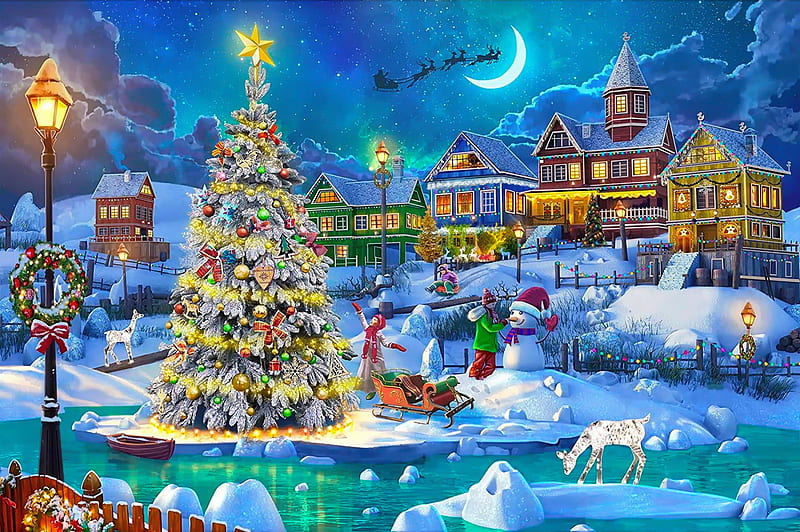In this animated illustration of a vibrant Christmas town, the scene exudes festive cheer amidst a winter wonderland backdrop. Dominating the left side of the image is a towering, fully decorated Christmas tree, resplendent with twinkling gold lights, a gold star perched on top, red ribbons, and an assortment of green and gold ornament balls. Resting on a substantial iceberg, this tree is accompanied by a small brown boat and a gleaming white and black reindeer figure. Nearby, a brightly lit streetlamp adorned with a festive green wreath, red ribbon, and red decorative balls brings an additional touch of holiday spirit.

The bottom left corner features a red fence, hinting at a cozy, homey scene, while icy patches and a cold, melting stream with reindeer standing on small islands traverse the foreground. Children in this lively vista are joyfully crafting snowmen and sledding, enhancing the scene's charm and warmth.

In the middle distance, classic Valley Victorian homes, in shades of brown, green, blue, and yellow, each bedecked with Christmas decorations and warmly lit windows, line the quaint town streets. Above this picturesque setting, the deep blue, cloud-speckled night sky hosts a crescent moon and the silhouetted figure of Santa Claus soaring through the sky in his sleigh, pulled by eight flying reindeer. This magical scene captures the essence of a heartwarming, storybook Christmas.